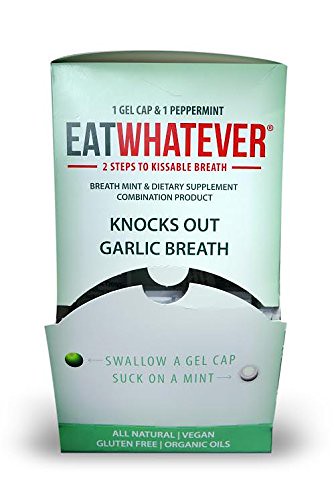This image showcases a close-up view of a small rectangular product package designed for easy access to individually wrapped servings of gel caps and mints. The packaging features a functional cutout at the front, allowing users to easily pull out the servings. The box itself has a gradient color scheme, transitioning from lime green or mint green at the top to a transparent background at the bottom.

At the top of the package, the text reads "One Gel Cap and One Peppermint" in small letters. Below that, the brand logo "Eat Whatever" is prominently displayed, with "Eat" in green and "Whatever" in red. Underneath the logo, the phrase "Two Steps to Kissable Breath" is written in small red letters. In the middle section, the text "Breath Mint and Dietary Supplement Combination Product" appears in small green letters, followed by a bold claim "Knocks Out Garlic Breath."

The bottom part of the package, where the opening is located, features instructions: "Swallow a Gel Cap" with an arrow pointing left towards an image of a small green ball, and "Suck on a Mint" with an arrow pointing right towards an image of a small white mint ball. Lastly, a green banner at the bottom declares the product's qualities: "All Natural, Vegan, Gluten-Free, Organic Oils." The entire package is set against a transparent background, highlighting its design elements.